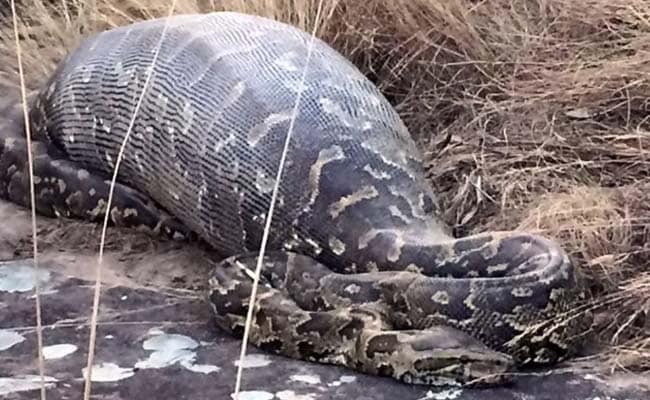The photograph captures a muted grayish-brown boa constrictor outdoors, lying partially on a grayish rock surface amidst yellowed, dead, and long grasses. The quality of the image is not very high, as it appears grainy and lacks crisp details. In the middle of the photograph, the snake's abdomen is visibly enlarged, indicating it has recently consumed a large animal. The snake's head, located in the bottom right corner of the image, and the tail section, are of normal size, while the midsection is notably distended. In the bottom left corner, three individual blades of brown grass extend from the bottom left to the top left of the image. The background is filled with brownish wild grass, adding to the natural setting of the scene. The snake's skin features lighter stripes running from its head to its tail.